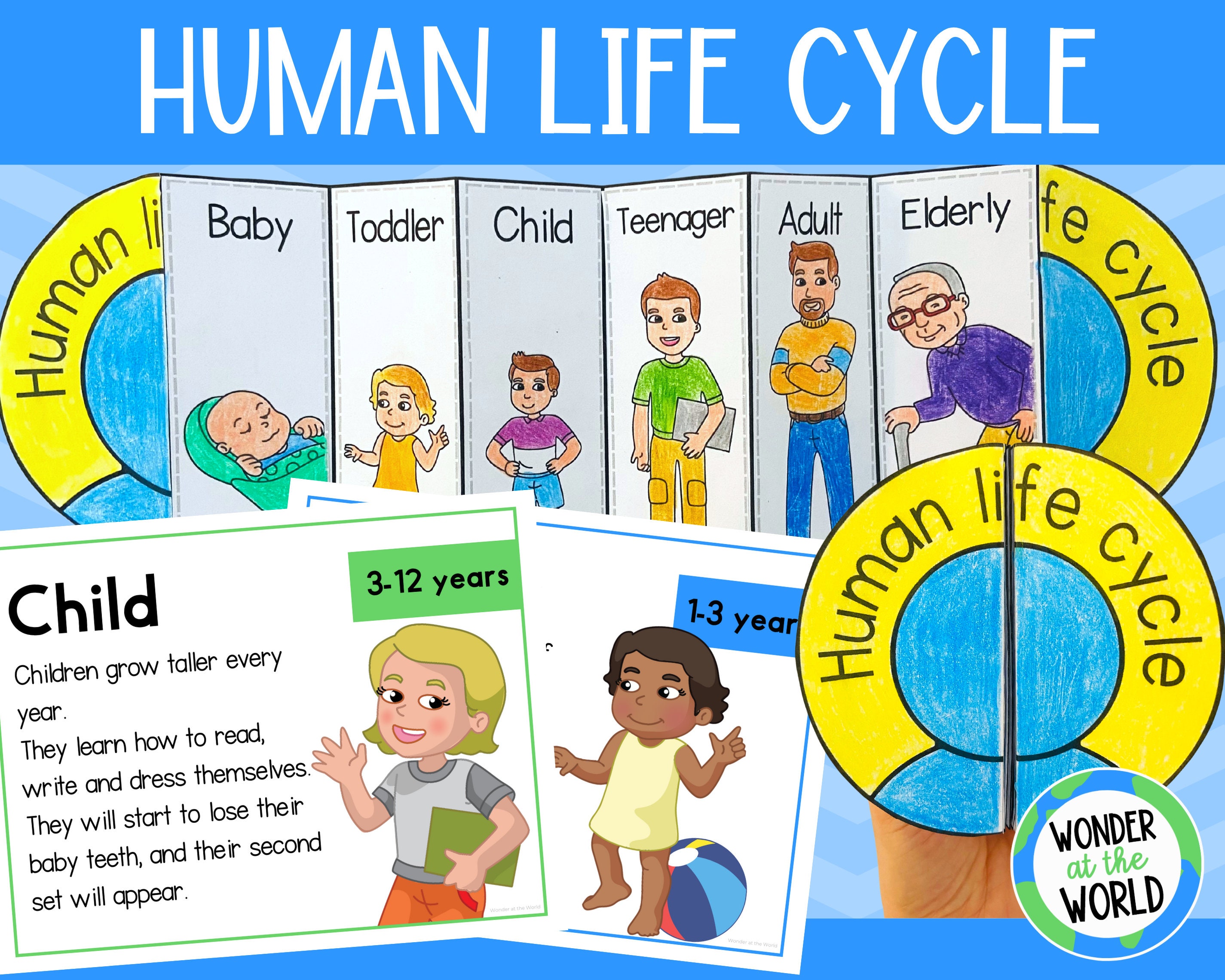The promotional poster is a rectangular image measuring approximately six inches wide and four inches high. It predominantly features a blue header at the top left-hand corner, spanning across the top and down about three-quarters of an inch, within which bold white text reads "Human Life Cycle." Below this header, there is a detailed fold-out pamphlet divided into several panels, each representing a stage in the human life cycle. These stages are labeled as Baby, Toddler, Child, Teenager, Adult, and Elderly, with a colored cartoon image depicting each age group.

The "Baby" panel displays a cartoon baby, while the "Toddler" panel has a child with yellow hair. The "Child" panel includes an image of a kid, and similarly, "Teenager," "Adult," and "Elderly" panels follow with respective illustrations. The Elderly illustration shows an elderly man with gray hair, glasses, a cane, and a purple shirt.

Extending from the left side of the pamphlet is a yellow banner inscribed with "Human, L.I.," which continues on the right-hand side of the fold-out to read "F.E. Cycle." On the lower right-hand side of the image, there's a blue circle with the surrounding yellow banner featuring the repeated text "Human Life Cycle." Additionally, a small white circle in the lower right-hand corner states "Wonder at the World," accompanied by a globe illustration.

Positional elements of the poster also include two white educational cards. The first card explains the "Child" stage, stating, "Children grow taller every year. They learn how to read, write, and dress themselves. They will start to lose their baby teeth, and their second set will appear," and it is accompanied by a picture of a child waving and holding a book, identified as a child aged 3 to 12 years, backed by a green background. The second card has a blue border with a white background and depicts a child aged 1 to 3 years.

Overall, the poster provides a visually engaging and informative depiction of the human life cycle through clearly marked stages and colorful illustrations.